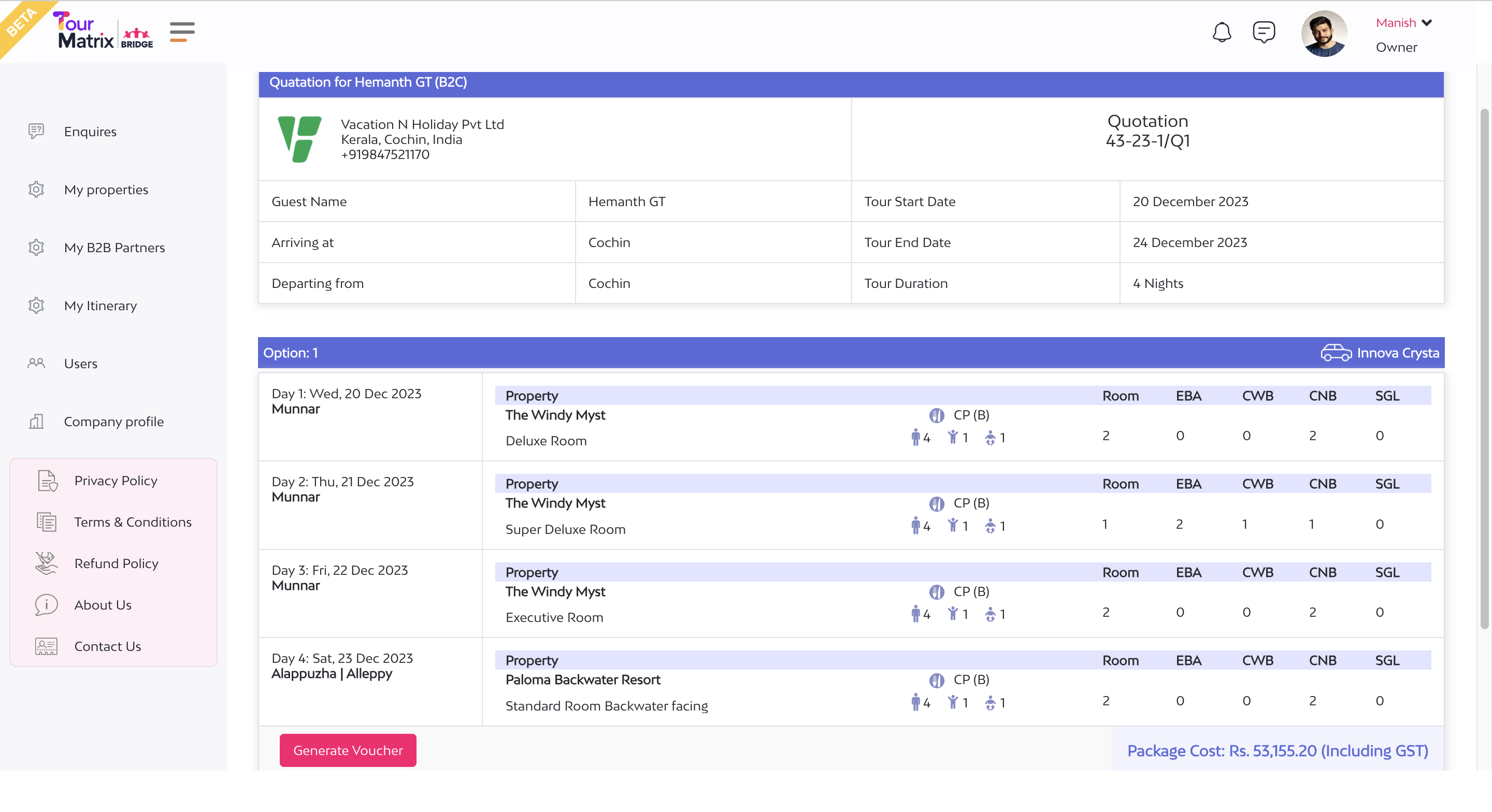The image is a screenshot of a webpage titled "Tour Matrix," currently in its Beta phase, as indicated by a yellow emblem in the top corner labeled "Beta." The interface prominently features a section labeled "Matrix" with an icon of people holding hands, all colored in pink. 

In the center of the screen, there's a green, uppercase "V" followed by the text "Vacation and Holiday Pvt. Ltd.", indicating it is an Indian company. Beneath this, the user's itinerary is detailed: the guest's name, arrival at Cochin, and departure from Cochin are all noted. 

The page then lists an "Action 1" section showcasing different properties and room options. Notably, two rooms are highlighted under "Windy Mist," although the exact location isn't specified. Users can choose from various room types including Deluxe Room, Super Deluxe Room, and Executive Room. Another property option is "Paloma Backwater Resort," which offers a Standard Room with a Backwater view. The webpage appears to have multiple sections, each detailing different property options for the user's booking preferences.